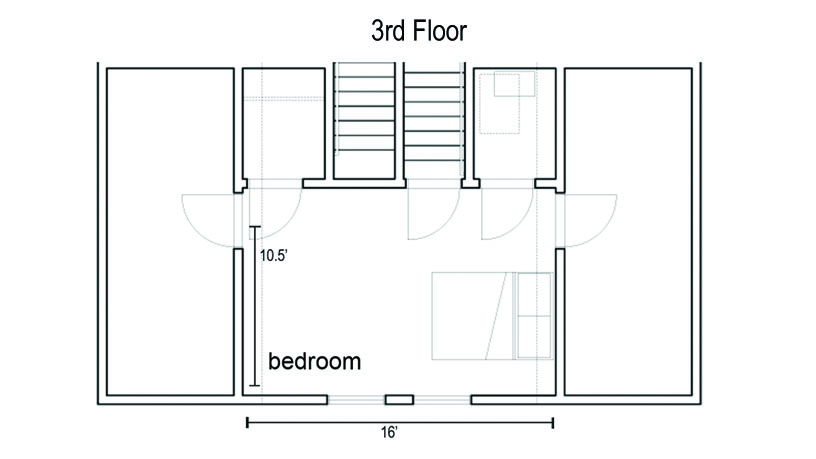The image depicts a meticulously drawn floor plan of the third floor, characterized by sharp, precise black lines and lighter gray details. The floor plan is rectangular, measuring 16 feet in width and 10.5 feet in depth. At the center of the floor plan is a room labeled "bedroom," which includes a light gray outline of a bed. Flanking the bedroom are rectangular areas to both the left and the right. Additionally, the plan features quarter-circle icons at various points to denote doors. At the top of the layout are two rectangular sections that are filled with horizontal, evenly spaced black lines, representing staircases. The bedroom is the only space shown with furniture, emphasizing the bed within the room.